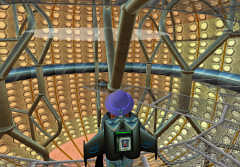A small, surreal image depicts a jet-fusion figure, with the body of a jet aircraft seamlessly integrated into the structure of a human. The jet, facing away from the viewer, has a person's head emerging from its top, although only the back of the head is visible. This enigmatic fusion stands on a transparent glass ledge, supported by a pipe-like framework, within a circular dome structure. Beyond the figure, there's a striking yellow globe, encircled by a pipe-like base at its midsection, adding a touch of industrial design to the scene.